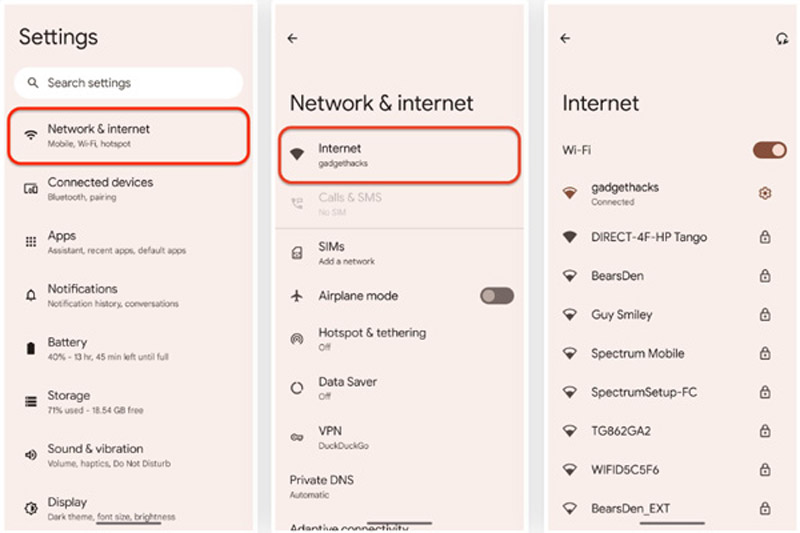This image features three sequential screenshots, arranged in three vertical columns, each capturing the steps of navigating through a device's settings. The screenshots share a peach-colored background.

**First Screenshot (Upper Left Corner):**  
The initial screenshot depicts the main settings menu. At the top, it displays the word "Settings" with a search bar beneath labeled "Search settings". The highlighted section, circled in red, is "Network & Internet." Below this selection are additional menu options: "Connected devices," "Apps," "Notifications," "Battery," "Storage," "Sound and vibration," "Display," and more.

**Second Screenshot (Middle Column):**  
The second screen focuses on the "Network & Internet" submenu. "Network & Internet" is also highlighted at the top. The term "Internet" is circled in red, indicating the subsequent selection. Below it are additional options: "Calls and SMS," "SIMs,” "Airplane mode," "Hotspot and tethering," "Data saver," "VPN," and "Private DNS."

**Third Screenshot (Right Column):**  
The final screenshot zeroes in on the "Internet" section, where wireless connections are managed. The "Internet" heading is at the top, with a toggle switch indicating that "Wi-Fi" is activated. The displayed list of available networks includes "Gadget Hacks," "direct-4f HP tango," "Bears den," "Guy smiley," "Spectrum Mobile," "Spectrum setup FC," alongside user tags labeled as someone's network, another user's network, and "Bears den extension."

Each screenshot is annotated with red markings to clearly guide the viewer's focus through the settings navigation process on the device.